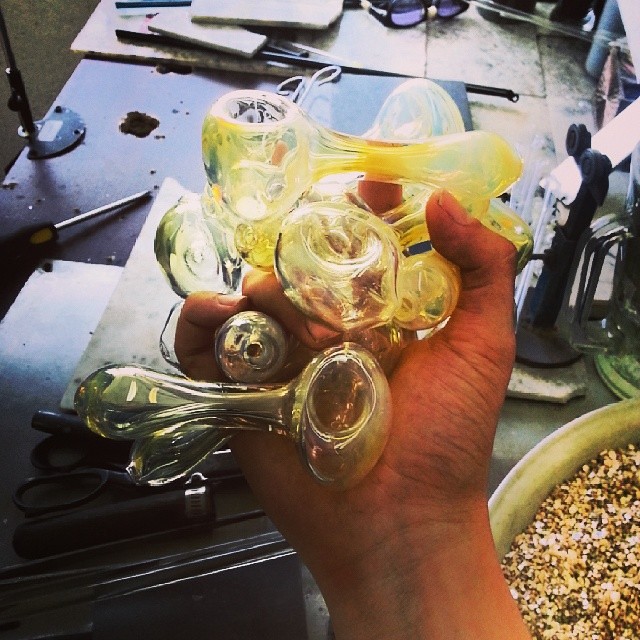In this overhead square photograph, a man's right hand is shown, palm up, clasping several intricate blown glass smoking pipes. His thumb and pinky are clearly visible, while the remaining fingers are obscured by the pipes. The pipes, numbering around six or seven, have distinctive deep bowls at one end for holding smoking material, combining clear glass and yellow hues. One of the pipes features a leafy design near the base, and the bowls vary in shape from circular to oval. The photograph reveals a cluttered black table in the background, scattered with several silver rectangular and circular objects, as well as a screwdriver indicating something is being disassembled. In the bottom right corner, there is a light green bowl containing various colorful, grainy seeds reminiscent of bird feed.